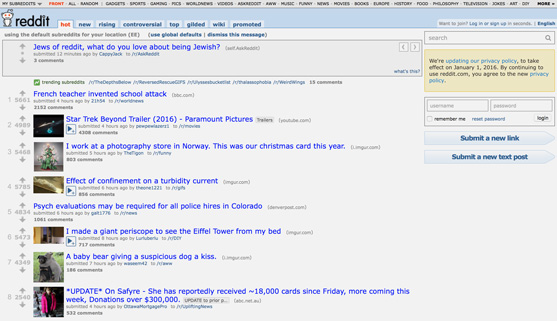This screenshot captures a classic "old Reddit" page, characterized by its nostalgic layout. At the very top, there's a classic menu stripe. Below that, the header is light blue and prominently features the Reddit logo alongside the word "reddit." Adjacent to the header are several navigational tabs.

This appears to be the homepage of "old Reddit." The leading section prominently displays a prompt titled "choose a Reddit," inviting users to share what they love about being Jewish. Just beneath this, some highlighted posts include intriguing titles such as "French teacher invented school attack" and "Star Trek Beyond trailer 2016," indicating the age of the content captured.

Throughout the page, all text is displayed in a clear, black font, while hyperlinks are distinctly blue, typical of the older Reddit interface. The background maintains a clean, white appearance, providing a stark contrast that enhances readability. Images are situated to the left of many of the links, adding a visual element to the list of posts.